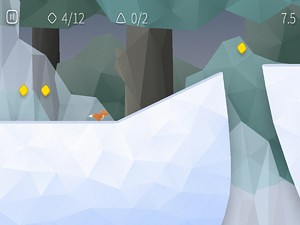The image appears to be a computer-generated still from a video game that features a geometric style reminiscent of Minecraft. Dominating the scene is an orange fox with a white belly and tail tip, running over a white, snowy, or icy ground. The fox seems to be navigating a landscape that includes a hill and a gap it must jump over to reach another white ledge.

In the background, primarily to the left, are clusters of brown tree trunks of varying shades and topped with green, triangular leaves, suggesting a forest setting. Additional greenery in varying shades of green appears on the right side. Large, white blocks resembling icicles or icebergs are also part of the scenery. The sky above is dark gray, adding a muted tone to the image.

The top of the image contains several infographics and numbers: "4 out of 12," "0 out of 2," and "7.5," likely indicating game statistics or objectives. There is also a symbol in the left corner that looks like a pause or menu button. The overall geometric and pixelated visuals, along with these game elements, reinforce the impression of a video game capture.